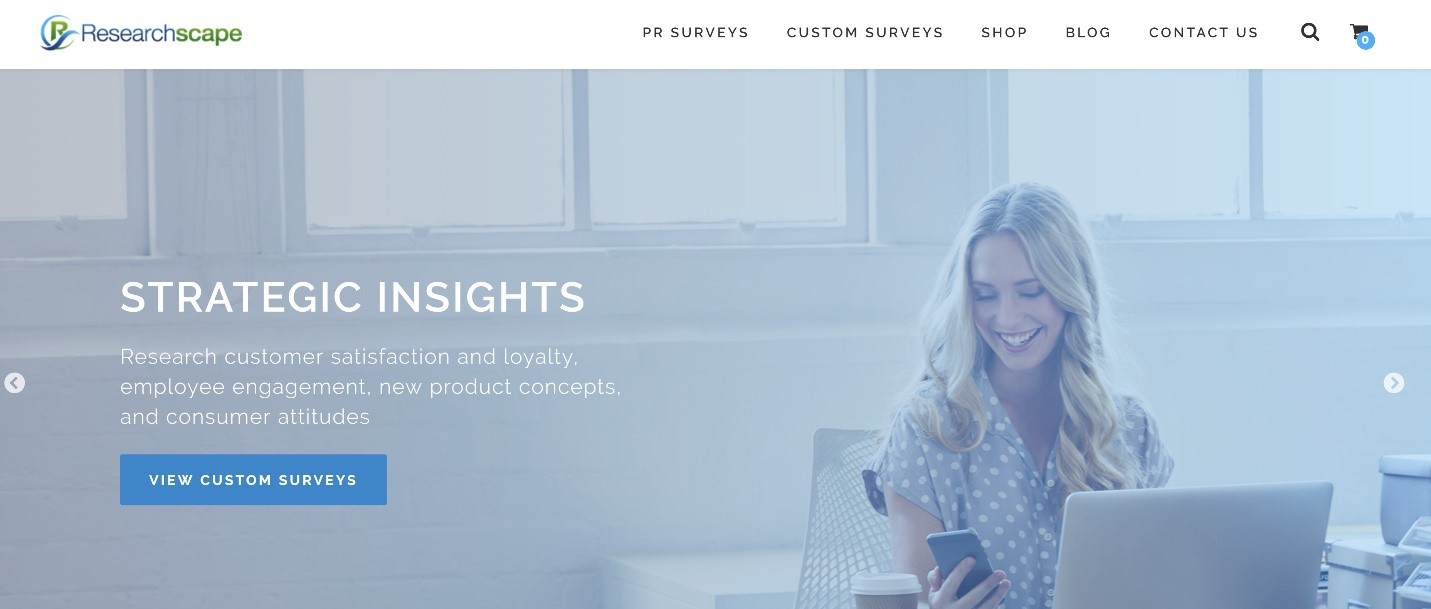The image is a rectangular, horizontally-oriented splash page serving as an advertisement or homepage for a business named "ResearchScape." The page features a smoky blue, almost hazy background. In the upper left corner, the company name "ResearchScape" is displayed alongside a logo consisting of a green "R" and an "S" within a blue circle, resembling a "C."

To the right of the logo, the navigation menu includes links labeled "PR Surveys," "Custom Surveys," "Shop," "Blog," and "Contact Us." Additionally, icons for a search function (depicted as a spyglass) and a shopping cart with a blue circle containing a white zero are present.

Beneath this header is a photograph of a smiling, blonde Caucasian woman. She is looking down and to her left at a cell phone she is holding in her right hand. The woman wears a white polka dot top, which appears slightly gray due to the bluish-gray background. She is seated in front of a laptop or computer monitor, and to the left of her, there is a brown beverage container with a white snap-on lid.

On the left side of the image, white text reads: "Strategic Insights, Research Customer Satisfaction and Loyalty, Employee Engagement, New Product Concepts, and Customer Attitudes." Below this text, a blue rectangle contains the phrase "View Custom Surveys" in white lettering.

The overall setting appears to be an office, inferred from the visible windows without curtains located behind the woman.